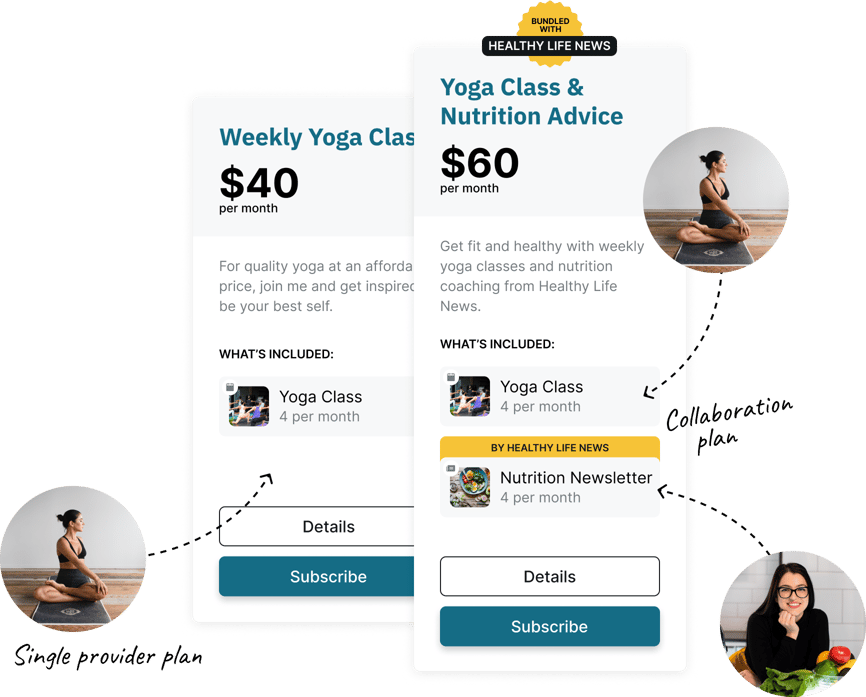The image is a screenshot of a promotional advertisement on a website. At the very top, the ad offers a bundle deal from "Healthy Life News" for $60 per month, which includes weekly yoga classes and a nutrition coaching newsletter. The headline reads, "Get fit and healthy with weekly yoga classes and nutrition coaching from Healthy Life News."

The ad details the package:
- **Weekly Yoga Classes**: Represented by an image of a woman practicing yoga, highlighted by a dotted arrow.
- **Nutrition Advice Newsletter**: Illustrated with a picture of a woman surrounded by vegetables, also highlighted by a dotted arrow.

Below these details are two buttons: a white "Deal Details" button and a dark blue "Subscribe" button.

In the background, there is a pop-up advertisement that offers a weekly yoga class for $40 per month. The headline reads, "For quality yoga at an affordable price, join me and get inspired to be your best self." This offer features the same image of the woman practicing yoga with a dotted arrow pointing to it. The plan is labeled as the "Single Provider Plan." This section also includes a white "Details" button and a dark blue "Subscribe" button.